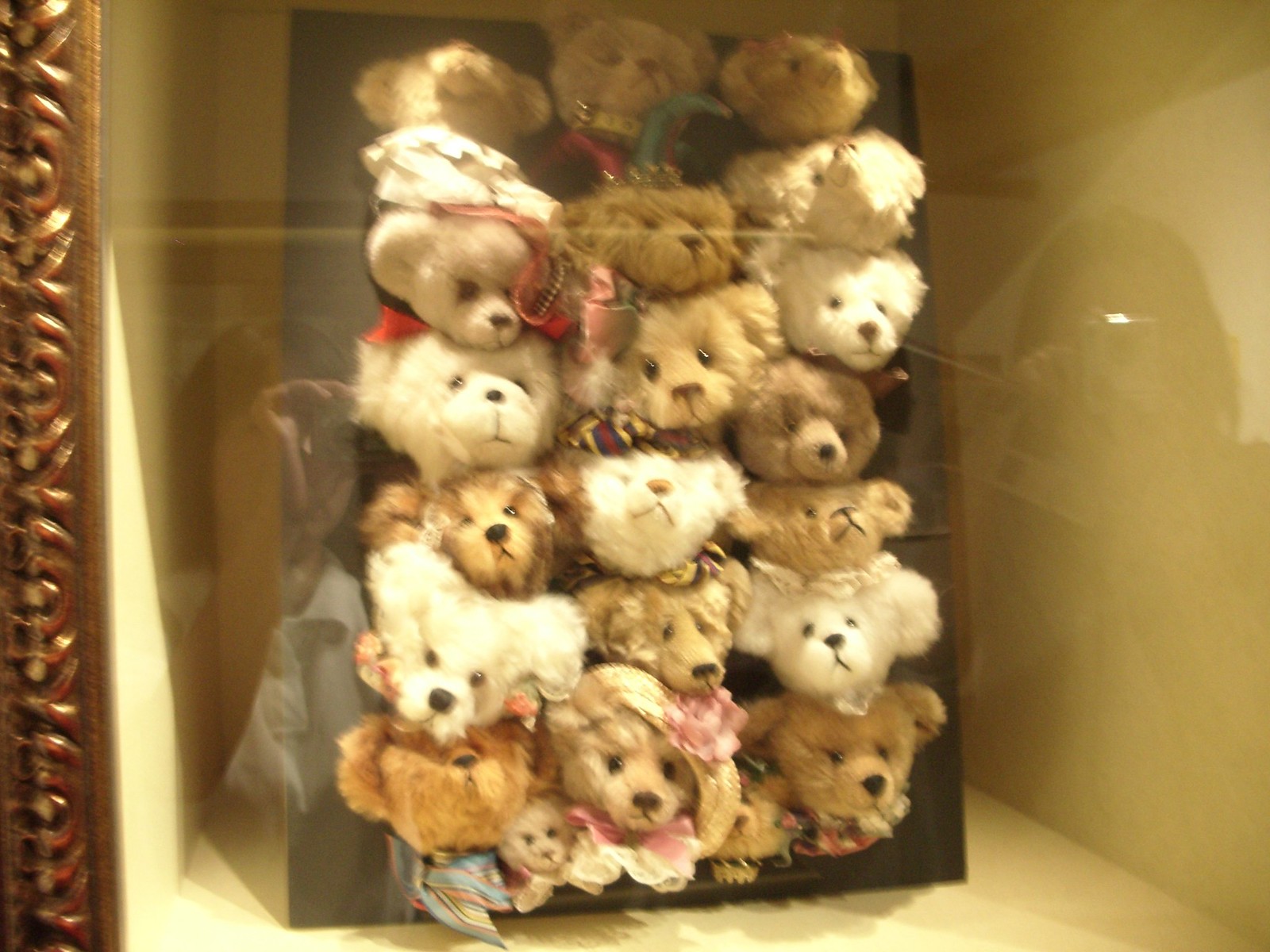The photograph depicts a detailed display of teddy bears arranged within a shadow box. The box itself, constructed of wood with an intricate gold-trimmed brown frame, appears to be fronted with glass, reflecting the photographer and another person standing nearby. The inside of the box is hollow with a mustard-colored interior, featuring a black rectangular background against which the bears are arranged. There are approximately 24 teddy bears, organized in six vertical rows and three columns, although a few rows divert from this pattern slightly. The bears are lined up so closely that only their heads are visible, with their faces pressed against the glass. They vary in color—mostly different shades of brown, tan, and white— and in size. Some bears sport decorative elements like pink bows, scarves, hats, or floral headpieces. The overall effect is of a charming, densely packed lineup of distinctly adorned teddy bear heads set against a carefully constructed and visually engaging backdrop.